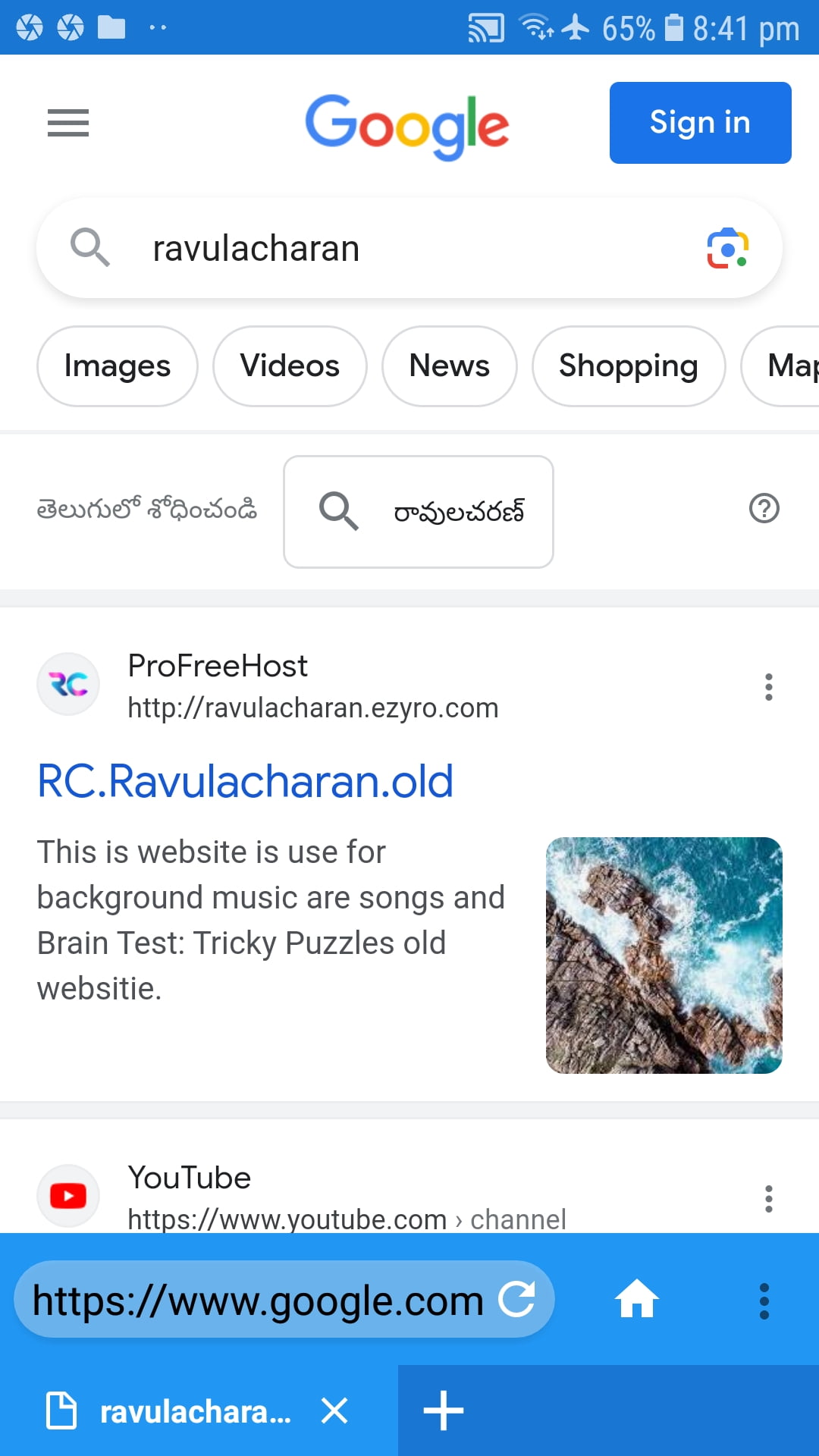The image features a predominantly blue interface with a multitude of icons and text. At the top, there's a solid blue bar. Within this blue bar are two light blue circles formed by angular triangle shapes, followed by an icon resembling a folder and two dots, all in light blue. Adjacent to these is an icon akin to a screen with a Wi-Fi symbol emitting from its side.

Further along, there's a depiction of a Wi-Fi symbol, an airplane icon, a '65%' battery indicator, and the time reading '8:41 PM'. The area below this bar is white, and features a grey triple-line menu icon positioned one above the other. The word "Google" is displayed in the brand's signature multicolored font. To the right is a blue rounded rectangle bearing the text "Sign In". 

Beneath this, there's a search bar containing a magnifying glass icon and the text "R-A-V-U-L-A-C-H-A-R-A-N", with a multicolored camera icon on the right. Below this text box, there are several grey rectangles with rounded edges, each representing different categories: "Images", "Videos", "News", "Shopping", and partially visible "M-A-P". Foreign characters follow these category tabs, along with another text box containing a magnifying glass icon and additional foreign characters.

Towards the bottom of the image, there's a grey circle outlined with a grey question mark inside it, a grey horizontal bar, and a grey circle displaying a small cluster of colors. This circle appears to contain the letters "R-C", though it is not entirely clear. Further text reads "Photo Free Host" with a web address "R-C-R-A-V-U-L-A-C-H-A-R-A-N dot old", and mentions the website is used for background music, R-songs, brain tests, and tricky puzzles, identified as an old website. An image of water and rocks is situated nearby.

Finally, there is a grey line and another grey circle encapsulating a red rectangle with an arrow pointing right, accompanied by the text "YouTube" and its related URL. The right-hand side of the image is populated with three vertical dots, followed by a blue rectangle. This blue rectangle contains a slightly rounded rectangle with the website name and a nearly complete circle, featuring an arrow at its top. Additionally, there's an icon of a house, another set of three stacked dots, an image resembling a piece of paper, the name "R-A-V-U-L-A-C-H-A-R-A dot dot dot", and an X. Concluding the image is a darker blue rectangle with a plus sign on its left side.